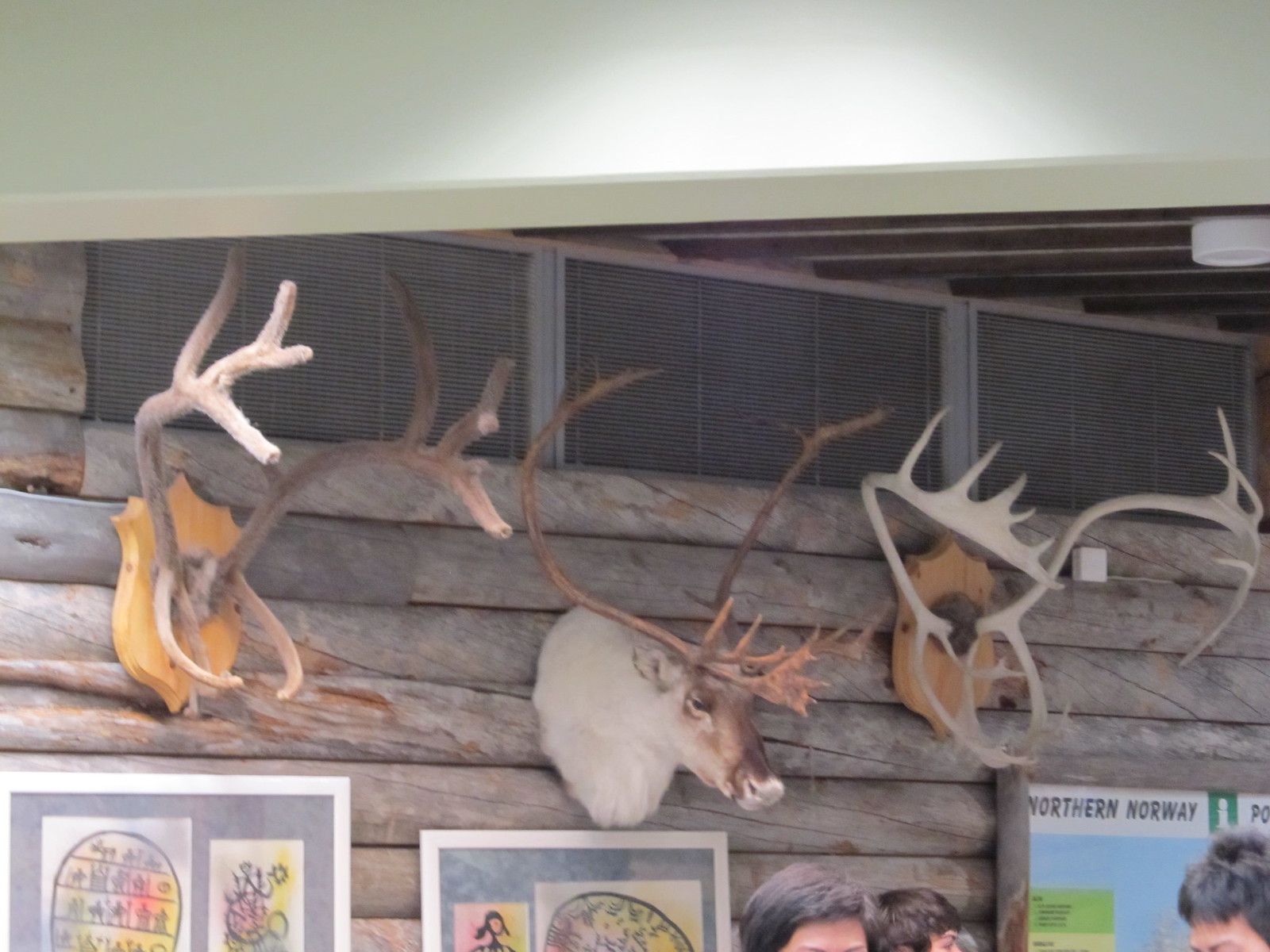In a rustic log cabin or lodge, a striking display of mounted wildlife adorns the wooden wall. Dominating the center is a majestic taxidermied white buck with an impressive set of large antlers. Flanking this central mount on both the left and right are wooden plaques, each showcasing even larger antlers that might belong to a moose, elk, or caribou. Below these mounts, only the tops of three heads with varying shades of brown and black hair are visible, adding a touch of human presence to the scene. Above, peculiar vents resembling a window punctuate the upper wall near the ceiling. Additional details include a plaque on the left side and signage on the bottom right reading "Northern Norway," along with some posters hanging below the human heads. The entire ambiance is steeped in a sense of rugged wilderness and traditional hunting lodge decor.